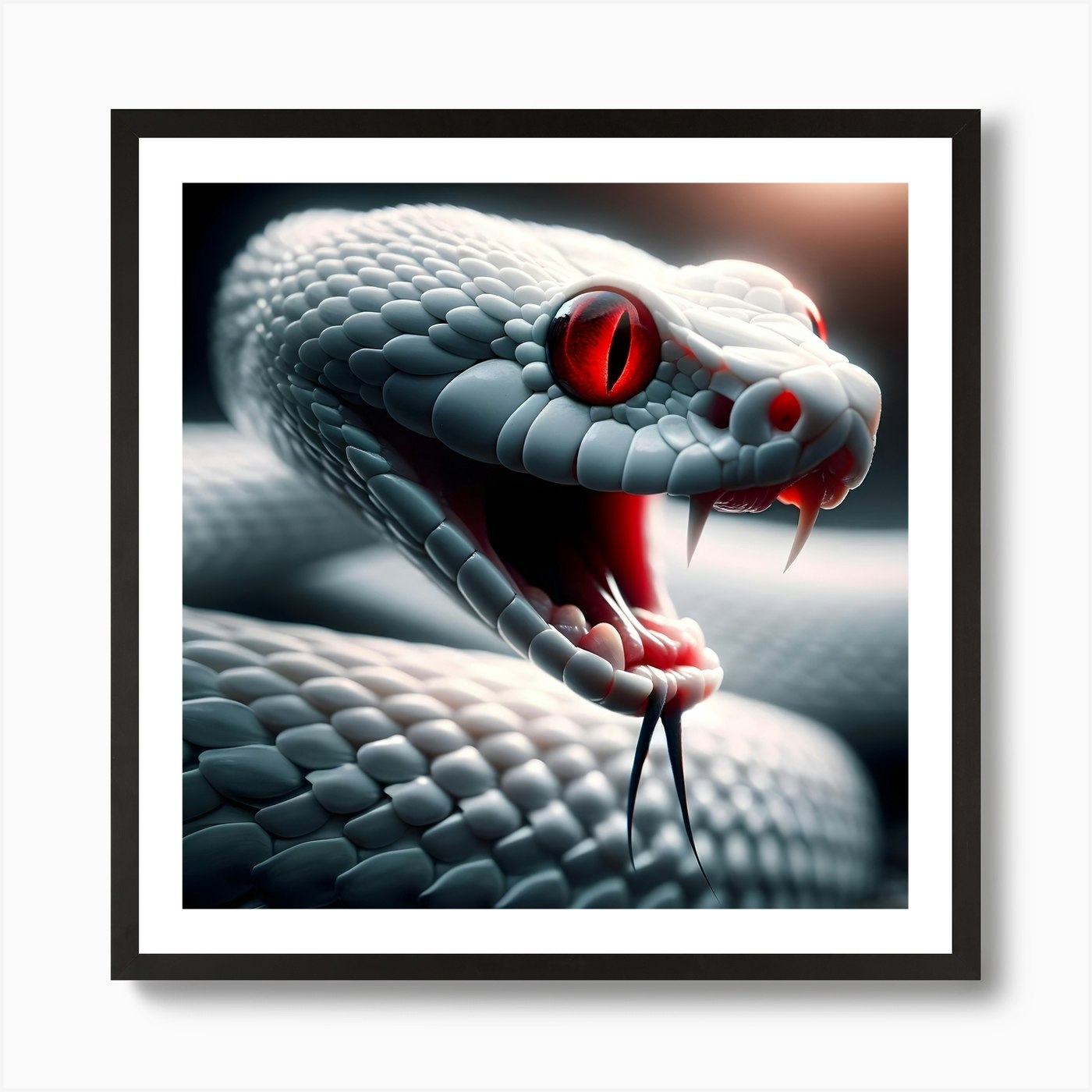This product photograph showcases a square poster beautifully rendered in 3D, framed with a sleek black border and a white inner edge. The centerpiece is a detailed depiction of a coiled, white snake against a seamless white void background, commonly used for online commercial purposes such as shops, catalogs, or websites. The snake is elaborately designed, with its body curled up and its head turned slightly to the right. The creature's fierce expression showcases its open mouth, revealing two prominent white fangs at the top and two black tendrils extending from the bottom jaw. The snake's red eyes, marked by black slits, stand out dramatically against the white scales, enhancing its menacing gaze. The lighting within this computer-generated image illuminates the interior of the snake's mouth and highlights the intricate details of its scales. Overall, this poster offers a striking visual, combining modern digital artistry with the classic elegance of a framed portrait.